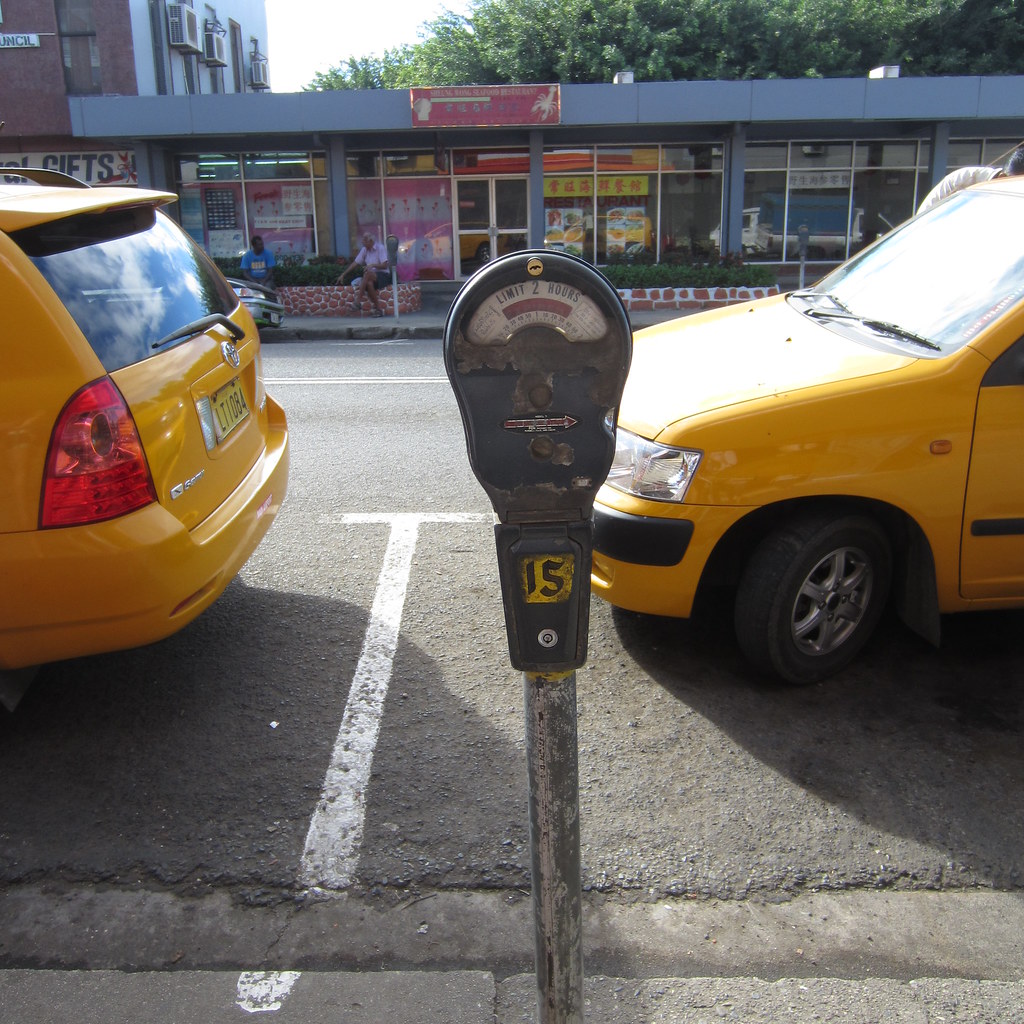The image depicts an old, rusted parking meter with the number 15 painted on it, positioned on the sidewalk beside a street. The meter features a small sign indicating a two-hour parking limit, with an arrow pointing right. Directly in front of the meter are two yellow cars, most likely taxis; one car is properly parked on the left while the other appears to be either poorly parked or in the process of parking, with someone conversing with the driver. The street itself is marked with white parking lines and two driving lanes. In the background, there is a row of stores. Some of the storefronts display Asian symbols, suggesting the location might be in Asia. The establishments include colorful signs and posters promoting products, with one shop specifically noted for selling gifts. Outside, a couple of people are seen sitting and chatting near two small garden pots. The scene is completed by the reflection of the yellow cars in the shop windows and a tree visible behind the buildings, adding a natural touch to the urban setting.